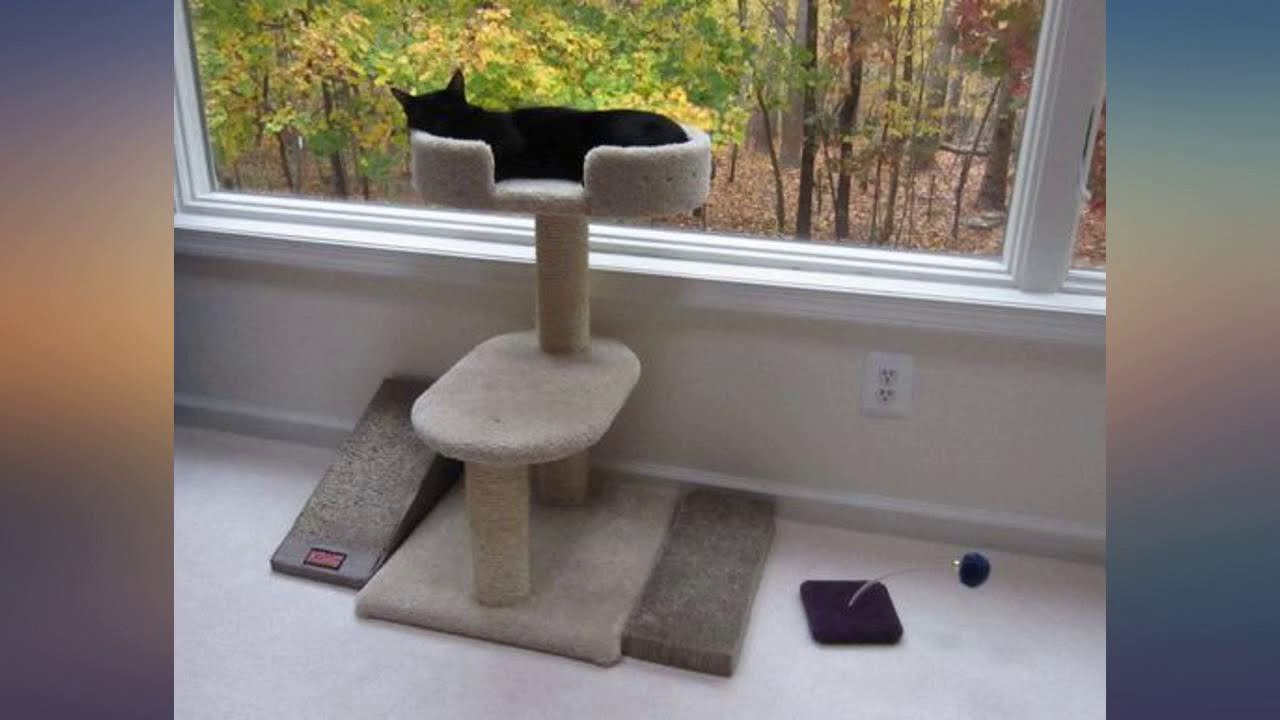In the cozy room of a house, situated in front of a large picture window almost reaching the floor, stands a light gray, three-tiered cat tower made of soft, carpeted material. Each level of the cat tower is supported by circular poles, with the base being a rectangular platform. The middle and top levels are uniquely shaped platforms positioned perpendicularly to each other. The window stretches the width of about three regular windows and is framed by white windowsills and separated by two vertical bars. The tower sits on a white floor, with a small slope on the left side and a darker gray rectangular board on the right. A purple cat toy with a fuzzy ball is also nearby.

Inside the top tier of the tower sleeps a black cat, comfortably nestled on the carpeted platform. Outside, the window reveals a picturesque wooded area in the midst of fall, exhibiting a spectrum of colors from magenta, yellow, and orange to green leaves. Though the sky is overcast, daylight softly illuminates the scene, casting gentle light on the rich tableau of autumn hues. The room itself has beige walls and gray carpet, complementing the serene and warm atmosphere of the space.